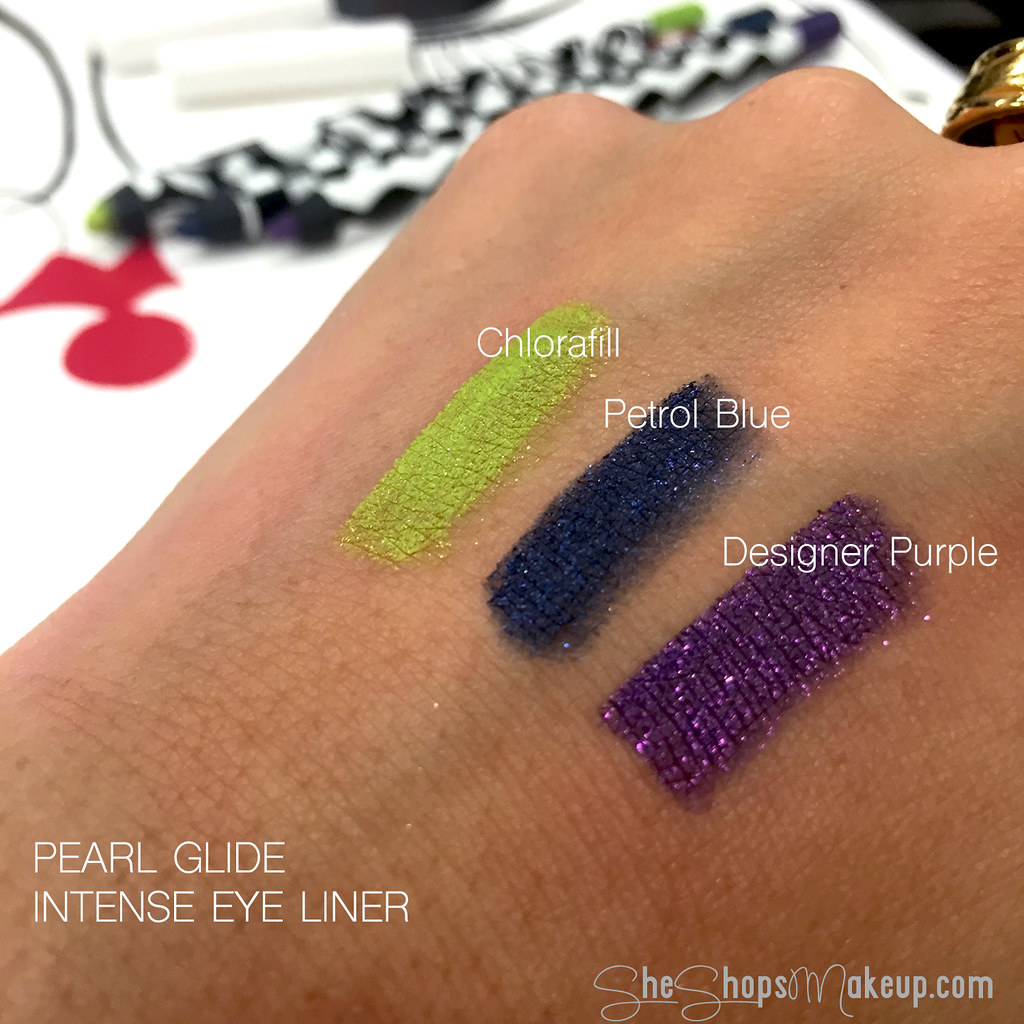This is a close-up photograph of the back of a white person's hand, showcasing three shades of Pearl Glide Intense Eyeliner for SheShopsMakeup.com. The shades are swatched on the right side of the hand: "Chlorophyll," a glittery green; "Petrol Blue," a deep navy with shimmer; and "Designer Purple," a sparkly dark purple. The background is mostly indistinct but features a red mark and a bag. The website SheShopsMakeup.com is displayed in the bottom right corner. The image combines product testing with a clear demonstration of the eyeliner colors and their glittery texture on a hand.